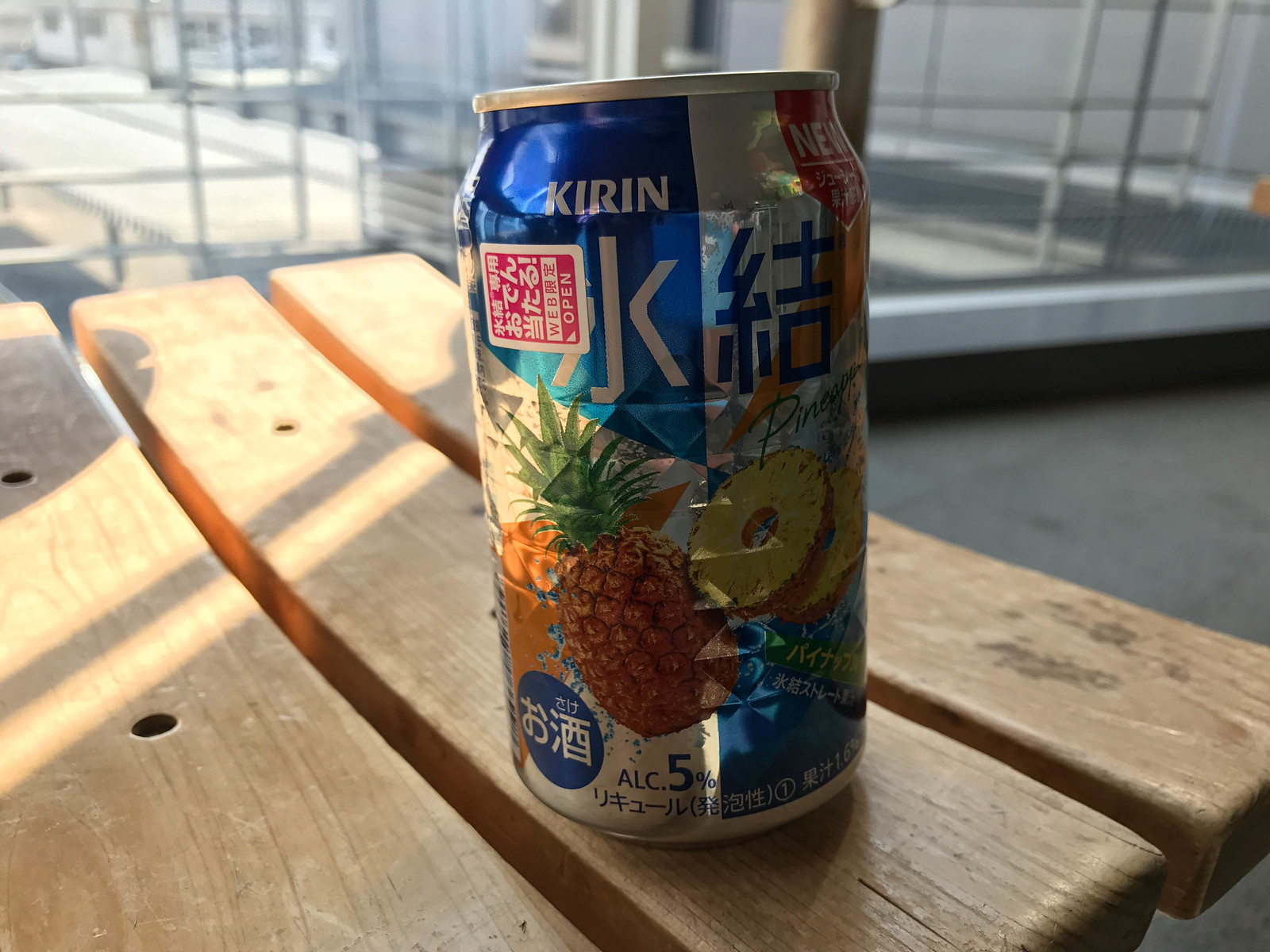This image captures a silver aluminum can, featuring vibrant colors and intricate designs, prominently displaying pictures of both whole and sliced pineapples. The can bears the brand name "Kirin" in the upper left corner, accompanied by various characters and symbols primarily in a non-English script. The text also includes "ALC 5%" indicating that it is an alcoholic beverage. Positioned on a rustic wooden bench or picnic table made up of three vertical planks with noticeable gaps between them, the can emits a tropical and refreshing vibe. The background is slightly out of focus, revealing blurry elements of a structure, possibly with windows or metal bars, and a concrete floor, adding a subtle urban touch to the setting.